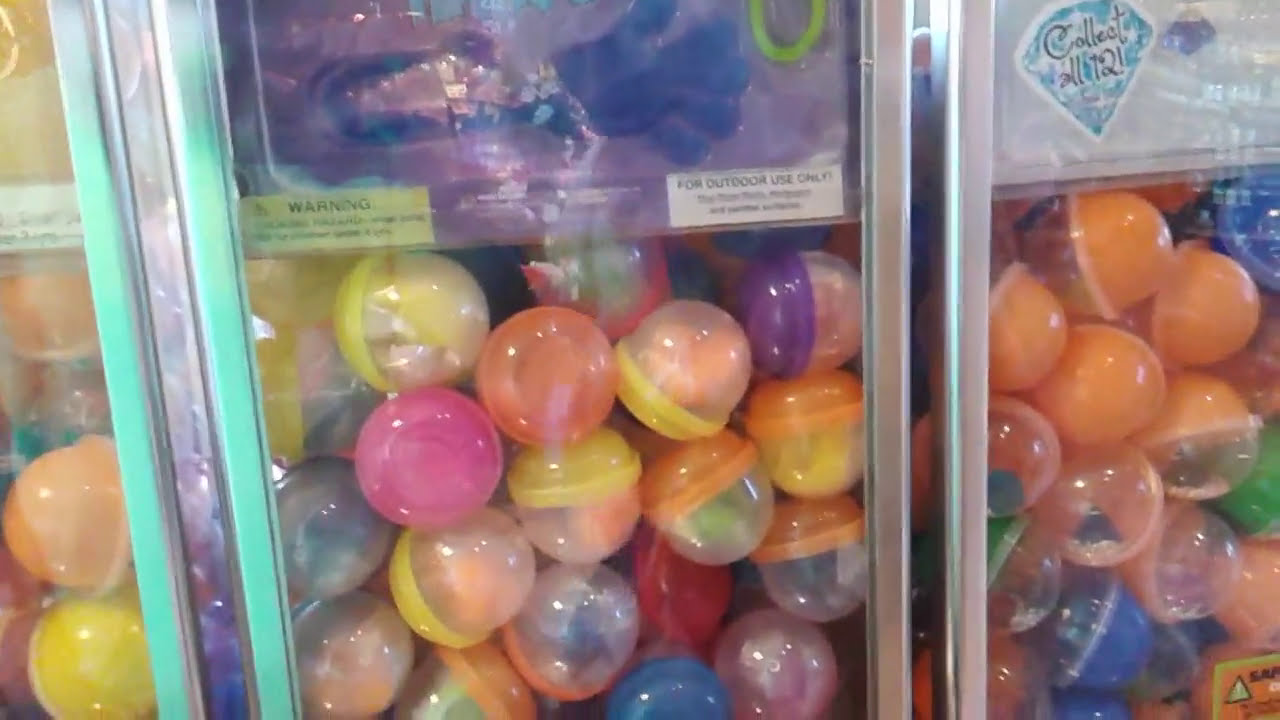This is a close-up, wide rectangular image showcasing three adjacent toy capsule vending machines, typically found outside stores or in shopping centers. The machines are made of glass and silver metal, each standing side by side. Only the central machine is fully visible, with the others partially obscured. The central machine prominently displays a stretchy, rubbery sticky hand toy, a popular novelty item for children. Below it are palm-sized clear plastic capsules with brightly colored lids in shades of blue, red, yellow, pink, purple, and orange, containing various toys wrapped in plastic. The left machine features solid yellow and orange containers while the right machine, also partially visible, has solid cups with clear lids and signage that reads "Collect All 12," indicating a series of collectible toys. The image is vibrant with bright, kid-friendly colors, emphasizing the playful and enticing nature of these vending machines.